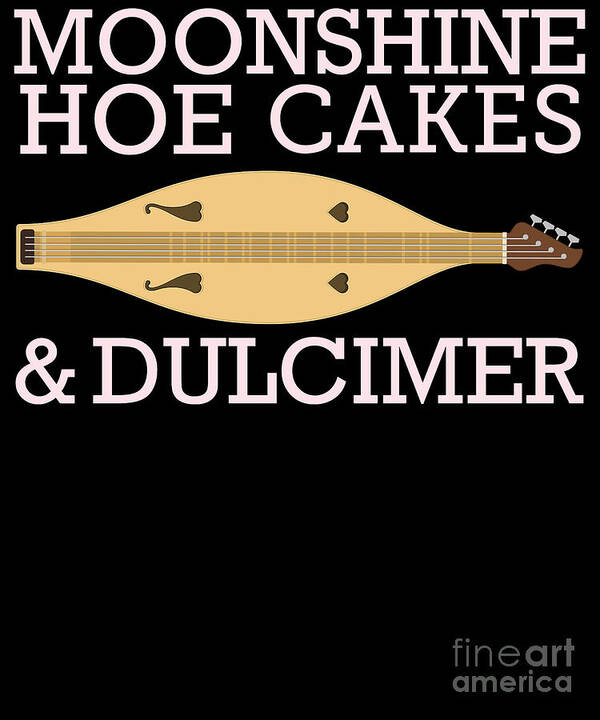The image is a vertically-oriented rectangular graphic featuring a predominantly black background. The lower half of the picture is almost entirely black, save for some notable text elements. At the top of the image, large white all-caps letters in a straight, blocky serif font read "MOONSHINE HOECAKES AND DULCIMER." Below this title is a cartoonish drawing of a stringed instrument, likely a dulcimer. The instrument has a beige oval body that tapers at the ends, a darker brown fretboard, and a headstock with four silver tuning pegs. The body of the dulcimer features heart-shaped sound holes. In the bottom right corner, there is a small gray watermark that reads "Fine Art America."